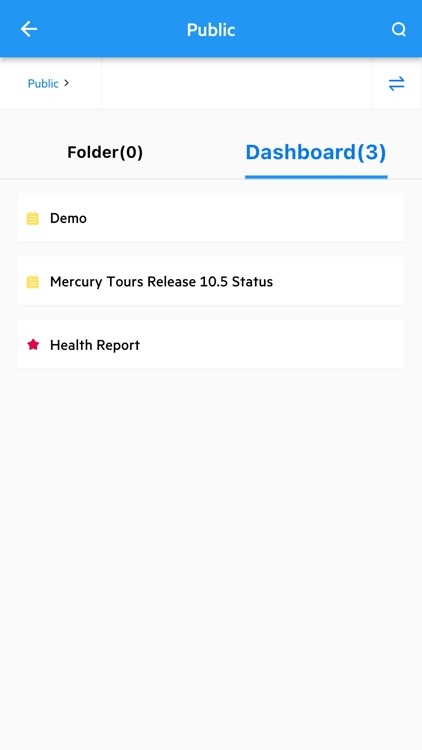This image is a mobile screenshot of an application interface. At the top of the app, a blue bar stretches across the screen. On the left side of this bar is a white back arrow, and on the right side, there's a white search icon. Centrally placed within the blue bar is the word "Public" written in white. Below this, on the upper left side, "Public" is repeated with a black arrow pointing to the right beside it. On the far right side, there's a blue filter icon.

The main background of the app is white, and just under the blue bar, two tabs are visible. The tab on the left is labeled "Folder," which shows it contains zero items. To the right, the tab labeled "Dashboard" is highlighted in blue, indicating it is active and contains three items. Below these tabs, the content of the "Dashboard" tab is displayed, which includes two folders and an item marked with a star. The first folder is titled "Demo," followed by another folder named "Mercury Tours Release 10.5 Status." The starred item at the bottom is labeled "Health Report."